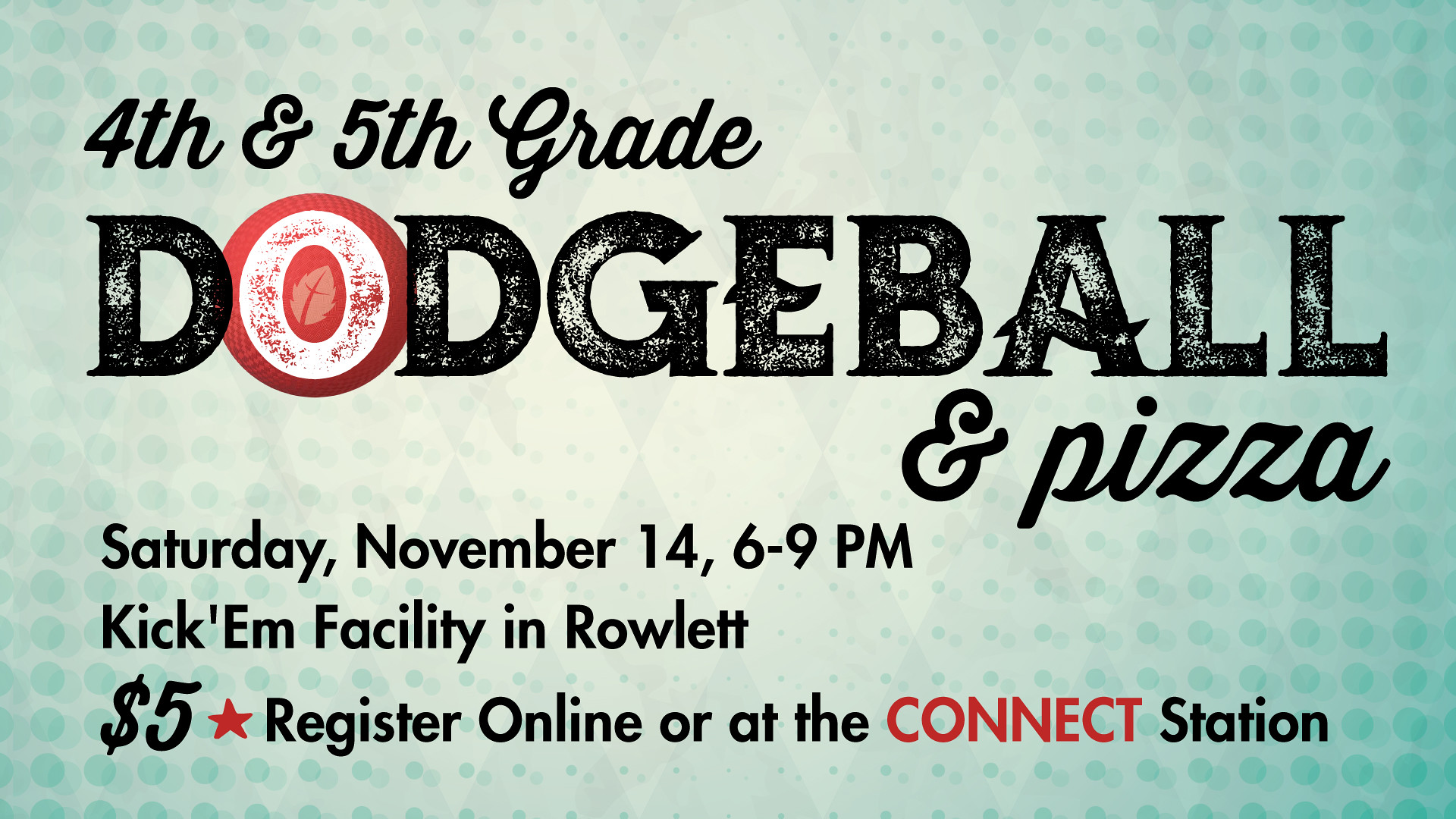This is a poster advertising a dodgeball and pizza event for 4th and 5th graders. At the top, in black script, it says "4th and 5th Grade." Below that, in large capital letters, it reads "DODGEBALL" with the 'O' in red. Right underneath, "Pizza" is written in cursive. The event details follow in black text: "Saturday, November 14, 6 to 9 p.m.," and beneath that, "Kickham Facility in Rowlett." Further down, it states "$5," with a red star between the "$5" and "Register," followed by the phrase "Register online or at the Connect Station" where "Connect" is in red. The poster has a teal, ombre-textured background with lighter polka dots of varying sizes that get smaller towards the center, lending a dynamic visual effect.